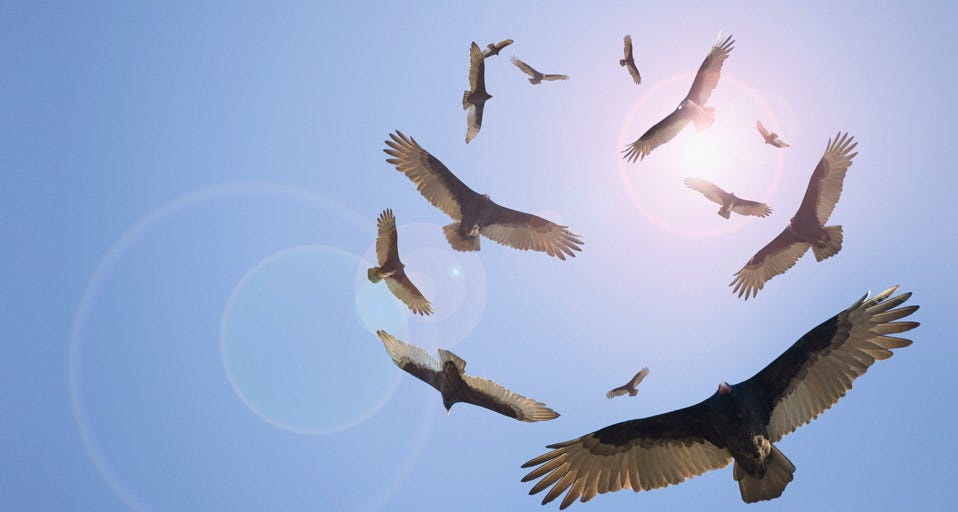This photograph captures a dramatic ground-up view of at least a dozen large scavenger birds, likely buzzards or vultures, soaring in a circular pattern against a clear blue sky. The image is horizontal and wide, emphasizing the birds as they appear to stack one over the other, ascending into the sky. Each bird is captured with outstretched wings, showcasing their characteristic black bodies and the distinctive grey or dull white feathers lining the edges of their wings and tails. The scene reveals the underside of the birds, highlighting their impressive wingspans and the small heads situated at the center of their expansive wings. The birds are primarily concentrated towards the right side of the photograph, giving a sense of organized motion as they follow one another in a spiraling formation, possibly in search of or awaiting the demise of potential prey below.